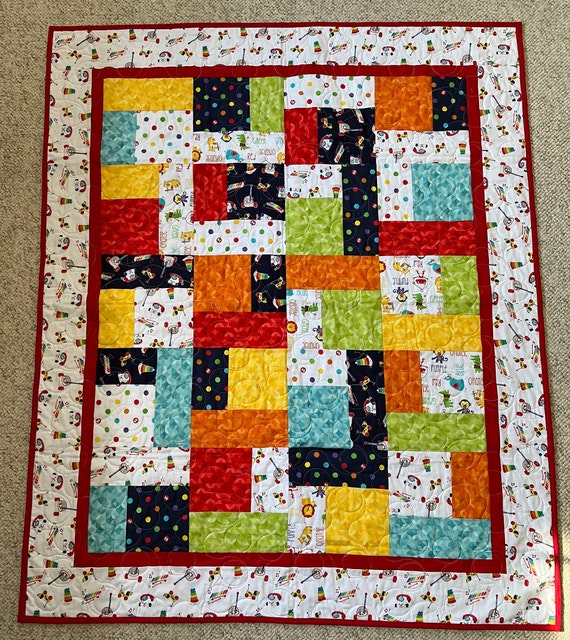The image showcases a large rectangular quilt or mat, set against a textured beige carpet, possibly in a residential setting. The background carpet has a threaded appearance with black flecks. The quilt features a detailed border and a vibrant mix of colors and patterns. Surrounding the quilt is a broad white border framed by two narrower red borders. The white border is decorated with images resembling children's toys in various colors. Inside the red-bordered area lies a colorful patchwork design, consisting of squares and rectangles in shades of turquoise, green, orange, yellow, and blue. Some patches use the same toy-themed material as the white border. Additionally, there are sections with polka dots on dark blue, white, and black backgrounds, showcasing colors like red, green, yellow, and orange, which are evenly distributed to maintain a balanced overall look.